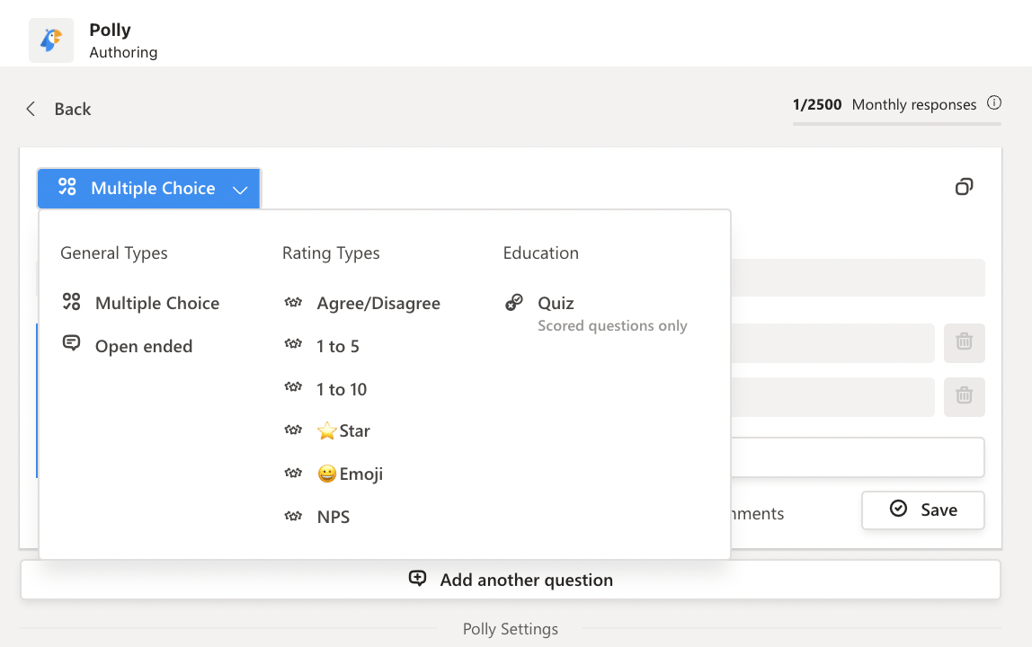A screenshot from a computer website features a detailed interface for a questionnaire or survey creation tool. In the top left corner, there is a square containing a cartoon drawing of a parrot with the label "Polly" and the word "Authoring" next to it. Below this header, a grayish-tan rectangle provides navigational and informational elements. On the left side of this rectangle, a "Back" button is displayed in black print. To the right, text indicates "1 / 2500 monthly responses."

Further down, the interface includes a section with several empty text boxes that users can type into, each accompanied by a trash can icon to delete the corresponding entry. Additionally, there is a save button with a checkmark icon for saving inputs.

Prominently overlaying this area is a blue rectangle labeled "Multiple Choice" that seems to offer various question type options. It lists categories such as "General Types," "Rating Types," and "Education." Under "General Types," options include "Multiple Choice" and "Open-ended." The "Rating Types" category offers scales such as "Agree/Disagree," "1 to 5," "1 to 10," "Star," "Emoji," and "NPS." For "Education," the available type is "Quiz." Three small circles and a checkmark symbol denote selection and interaction options within this section. Overall, the image provides a comprehensive view of the survey tool's layout and functionality.